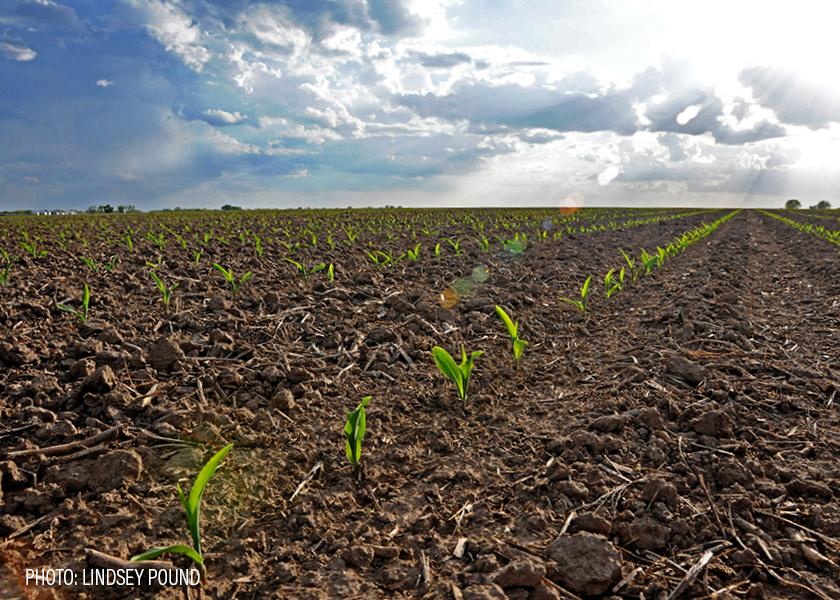The image captures an expansive agricultural field under a blue, partly cloudy sky. The field is filled with rows of dark brown soil, each row neatly lined with small green plants sprouting up, likely young corn seedlings. The camera angle is ground-level, emphasizing the orderly rows that stretch into the distance. Small rocks, twigs, and clumps of dirt are visible between the rows. The sky above features fluffy white clouds with patches of blue, transitioning to darker shades towards the left. Sunlight filters through the clouds, creating rays that illuminate the scene. In the background, a few green trees border the horizon. A bright spot in the upper right corner highlights the sun. At the bottom left corner of the image, the text reads, "Photo: Lindsey Pound."